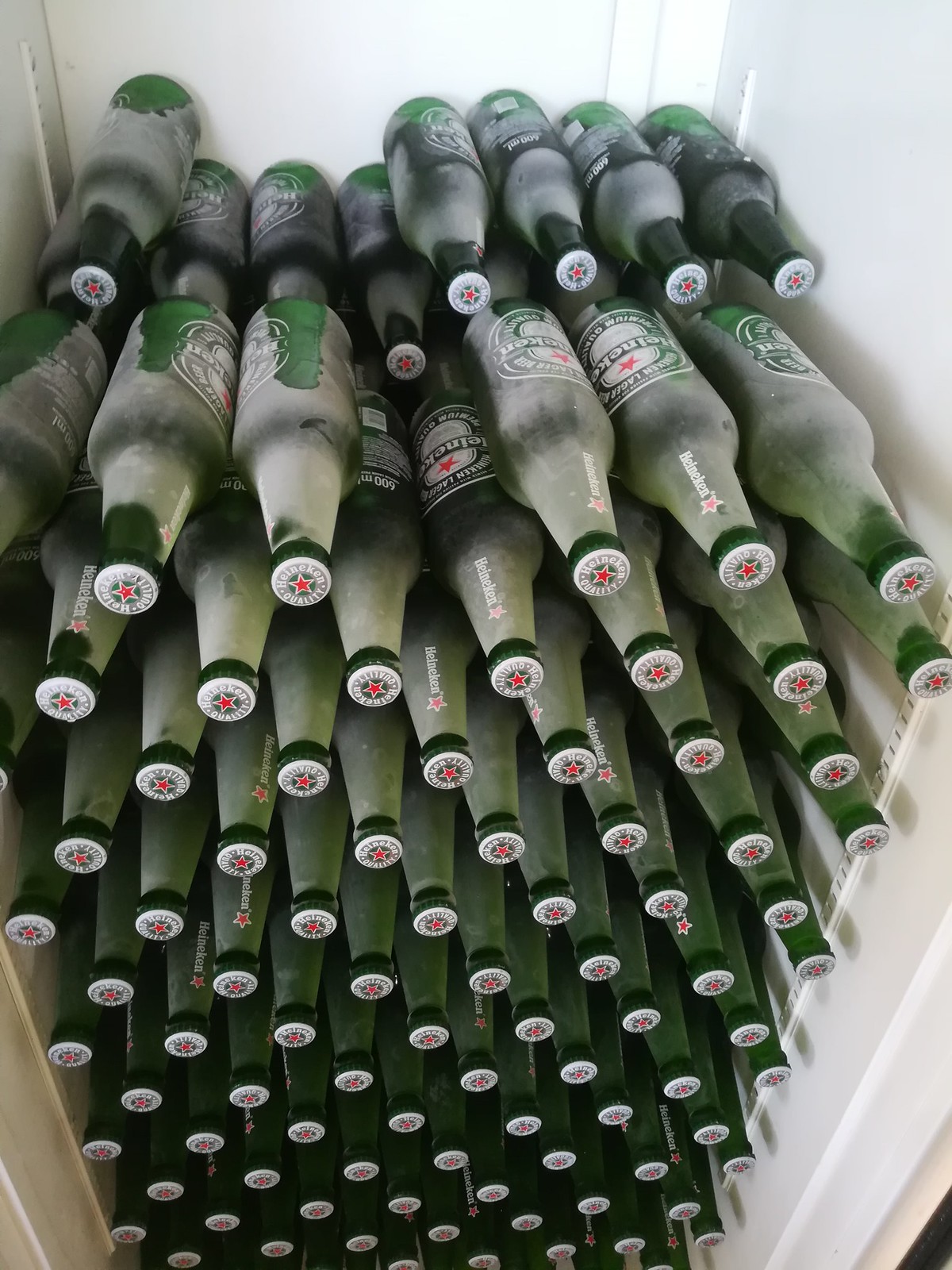This image depicts the interior of a vertical, white, plastic-lined refrigerator, densely packed with approximately 100 frosty Heineken beer bottles. Arranged meticulously in two stacks, one in front of the other, the green bottles cover the entire inside space, stretching from the bottom to almost the top of the fridge. Each bottle is recognizable by its classic white label with the iconic red star above the green Heineken logo, also mirrored on the white caps with red star detailing. The distinct light frosting coats most bottles, suggesting they are well-refrigerated, adding a whitish hue that overlays the green glass, with some areas still revealing the original green color.